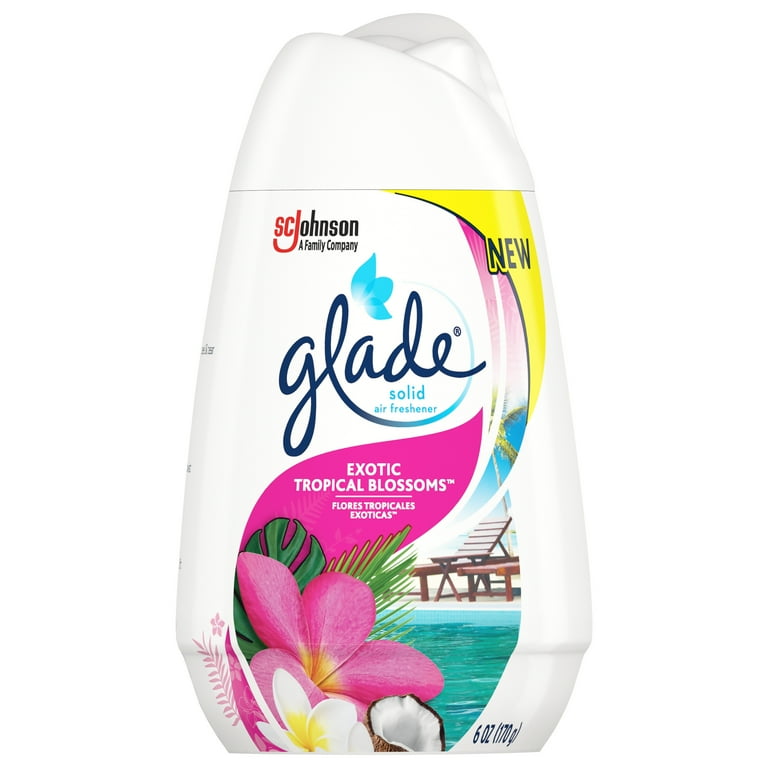The image is a detailed color photograph of a Glade solid air freshener container, in portrait orientation, against a white background. The container is made of white plastic, featuring a contoured, slightly pyramid shape that is narrower at the top and wider at the bottom, with a lid seamlessly integrated into its design. At the top left, the SC Johnson logo is displayed in red and black, accompanied by the phrase "a family company." On the upper right, the word "NEW" is prominently printed in bold black text.

Centrally positioned in dark blue script is the brand name "Glade," with a blue flower motif extending from the 'A' to the bottom of the 'L.' Below this, in small blue letters on the right, it identifies itself as a "solid air freshener." Beneath this text, a dark pink teardrop-shaped swash contains the white text "exotic tropical blossoms," emphasizing the scent. The bottom part of the container showcases a colorful illustration featuring several pink and white hibiscus flowers alongside a half-cut coconut, with a beach poolside scene with brown reclining chairs by an aqua pool to the right. The overall style of the photograph is representational realism, focused on product showcasing.